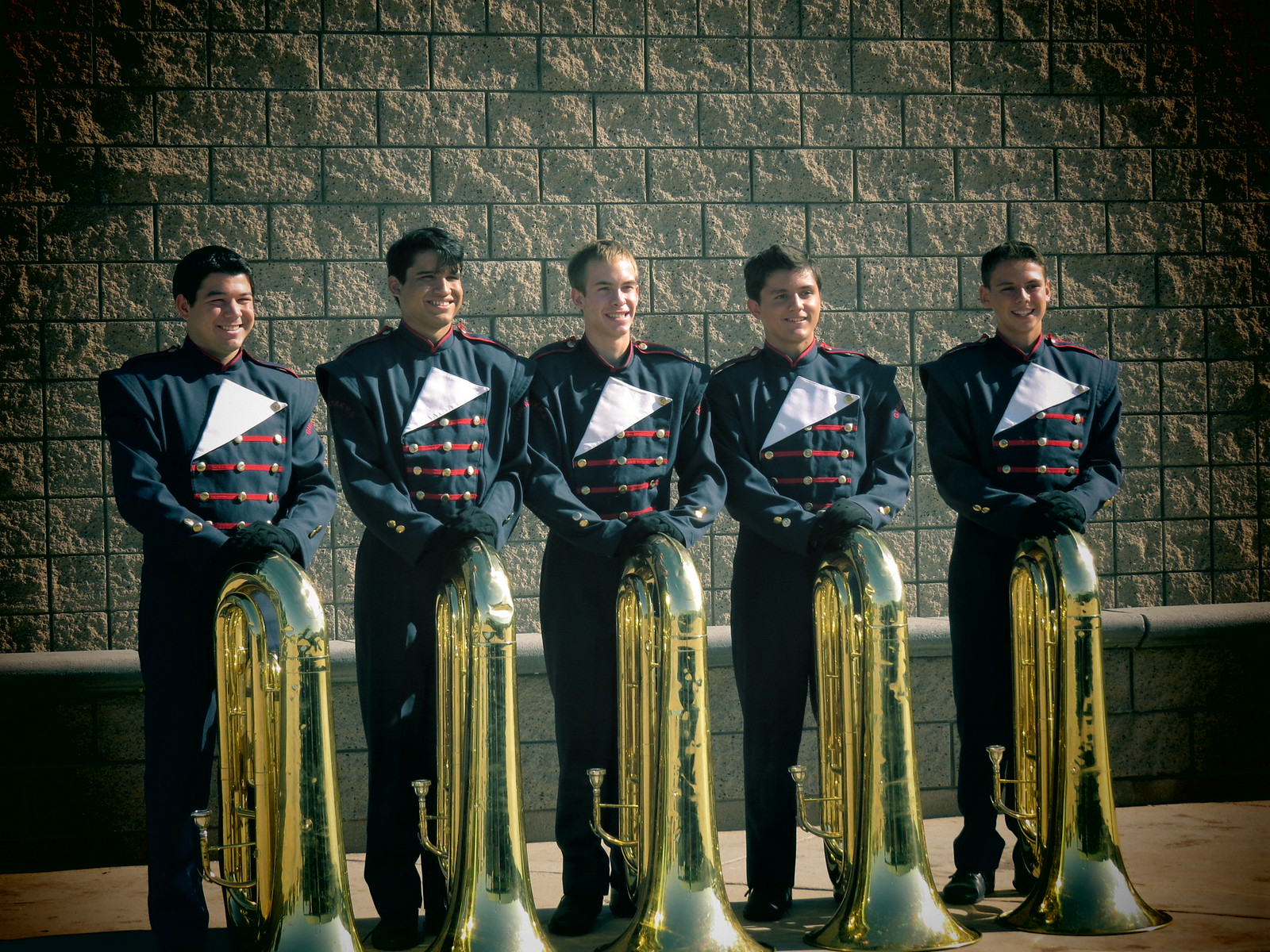In the image, five male band members are standing in a line on a cement floor, each holding a golden tuba, which rests on the ground with their hands on top. They are all dressed in matching dark blue band uniforms adorned with red stripes and gold buttons running horizontally across the chest, complemented by a distinctive white triangle on the chest. The backdrop behind them features a brown brick wall with a concrete lining at the bottom. The boy on the far right has short, greased-back black hair and a smile with a shadow cast on the left side of his face. Next to him is another smiling boy with black hair held up in the middle by mousse. The center band member, who also smiles, has short light brown hair. The tallest stands fourth, distinguished by longer black hair partially covering his forehead. The final boy on the far end sports short black hair and a round face.